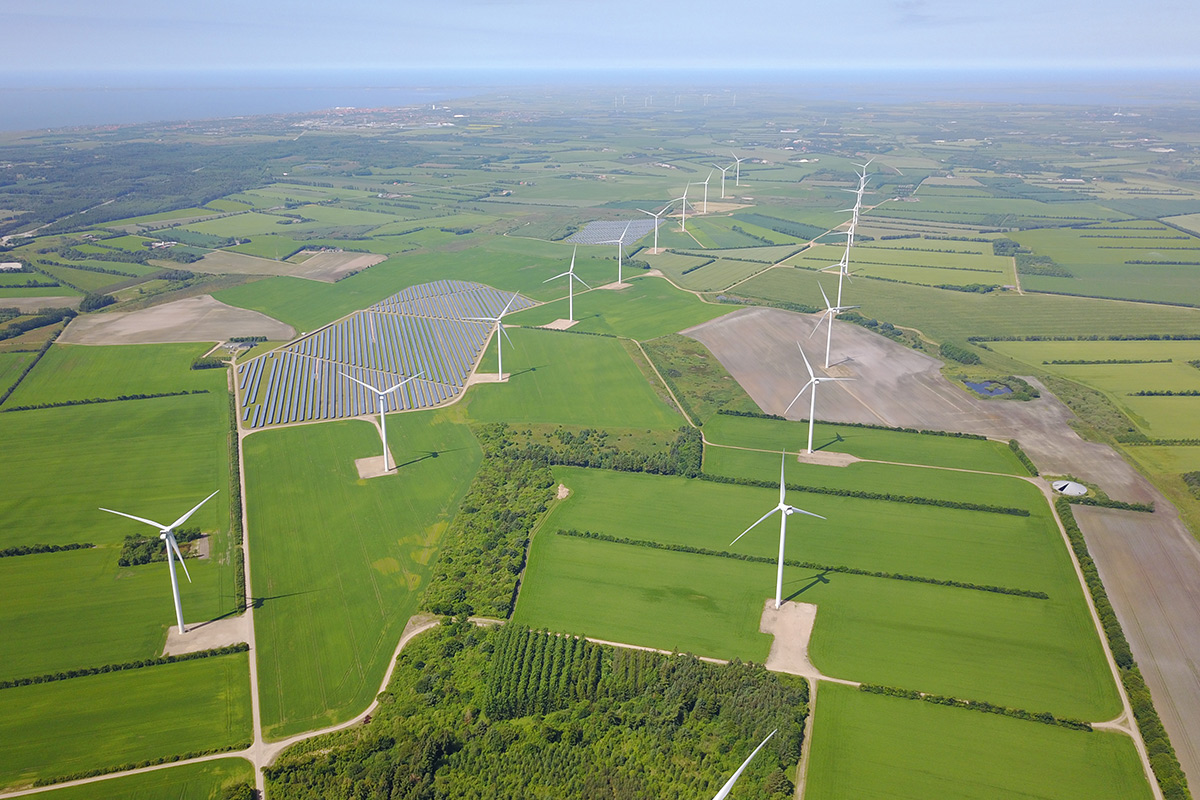Aerial view capturing a vast wind farm spread across green farmland with two distinct rows of white wind turbines stretching off into the distance. Each row contains approximately ten turbines, standing tall on patches of bare dirt with access roads leading to them. Interspersed among the turbines are a few plots—three or four—of solar panels. The landscape is largely free of crops, dedicated almost exclusively to these renewable energy installations. The horizon is misty, blending into a white sky. In the background, there are traces of water and darker, blurred areas, adding to the expansive and serene atmosphere of the scene.